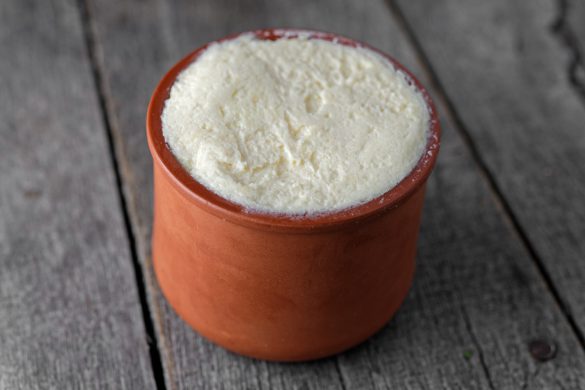The image depicts a small, reddish-orange ceramic bowl with no handle, similar to a clay ramekin, positioned on an aging, unfinished wooden picnic table with distinctive separations between the boards and visible rusty nails. The bowl contains a white, creamy, and slightly pasty substance that could be mashed potatoes, couscous, butter, cream cheese, or another similar material. Some of this creamy substance has slightly overflowed and is smeared around the top edge of the bowl. The table, characterized by its grayed and weathered appearance, enhances the rustic ambiance of the scene.